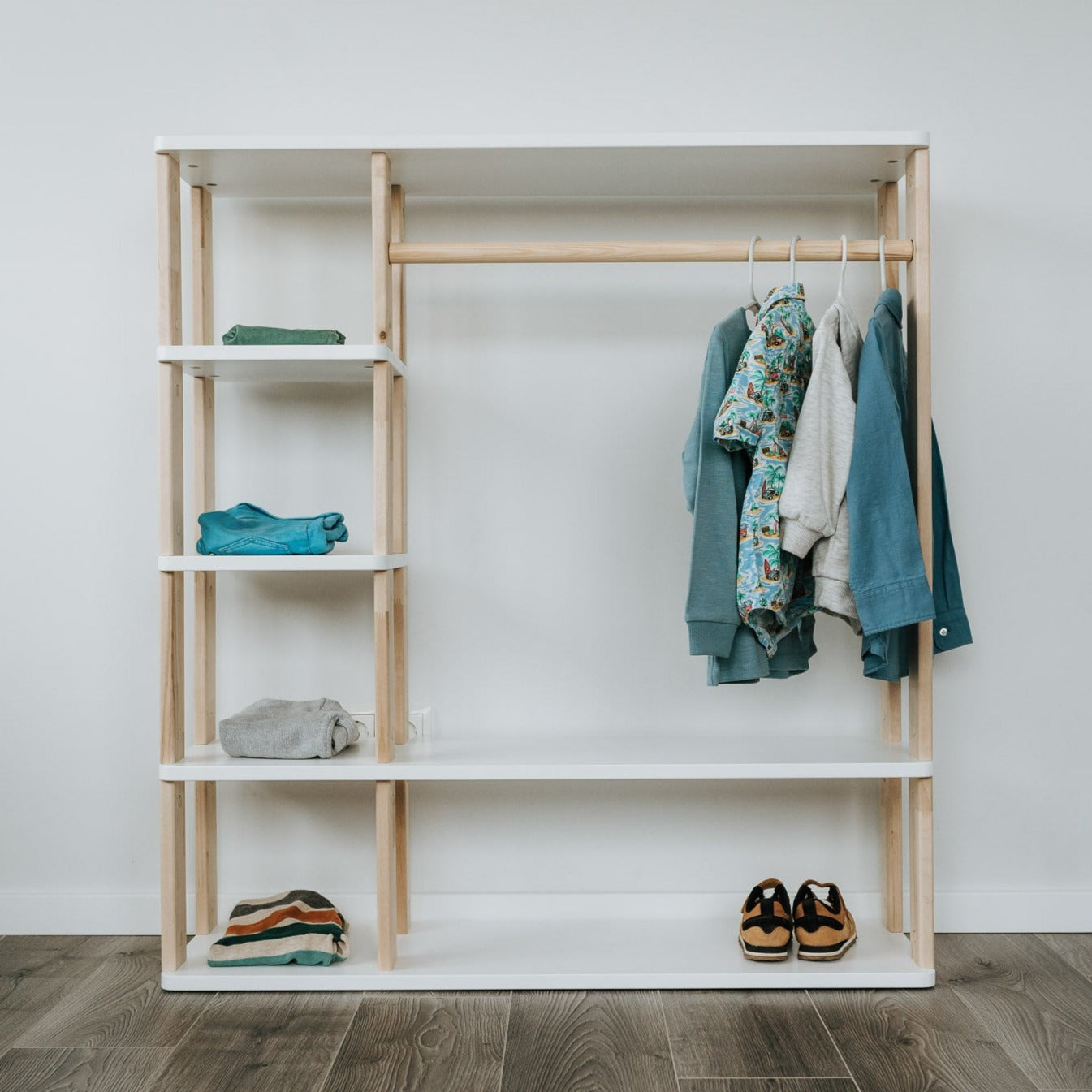This photograph showcases a versatile, stand-alone modular storage organizer, designed optimally for closet or bedroom use. The unit features a white frame accented with light pine wood posts, set against a white back wall and positioned on a grayish hardwood floor. The left side of the organizer includes three small shelves, each with neatly folded clothing: a green shirt on the top shelf, blue jeans on the middle shelf, and gray sweatpants on the lower shelf. The bottom-left section also holds a striped shirt. On the right side, a wooden rod supports an array of hanging items such as jackets, hoodies, and a dress shirt. Below the hanging rod, the bottom shelf houses a pair of brown shoes on the right side. The minimalistic and functional design of this modular shelving provides ample storage solutions while maintaining a clean and organized appearance.